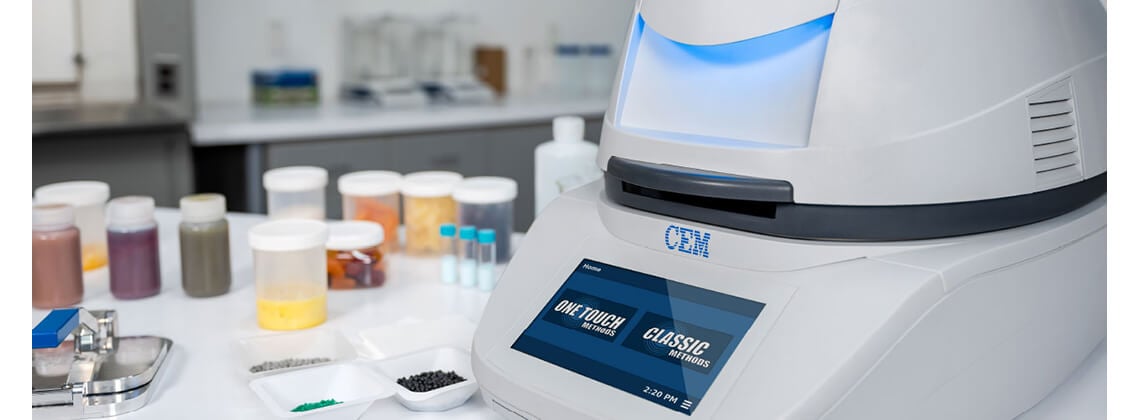This image depicts a wide, white table within a laboratory setting, possibly a biological or chemistry lab. Dominating the right side of the foreground is a white piece of machinery fitted with a blue touch screen. This device, branded with the blue text logo "C.E.M.," prominently features the phrases "One Touch Methods" and "Classic Methods" on its front panel, alongside a visible timestamp. The machine has a lid for access and a vent for airflow.

Next to the machine, a variety of white bowls and containers are neatly arranged, holding substances that range from a black pepper-like material to silverish and bright fluorescent green powders. Additional waybouts filled with beads or powders can be observed. There is also a noticeable metal contraption with a blue handle nearby.

In the background, the laboratory extends with benches lined with additional scientific equipment, including scales. Transparent canisters that reveal variously colored powders or solid items are also scattered around, adding to the array of scientific tools and materials present in the workspace.